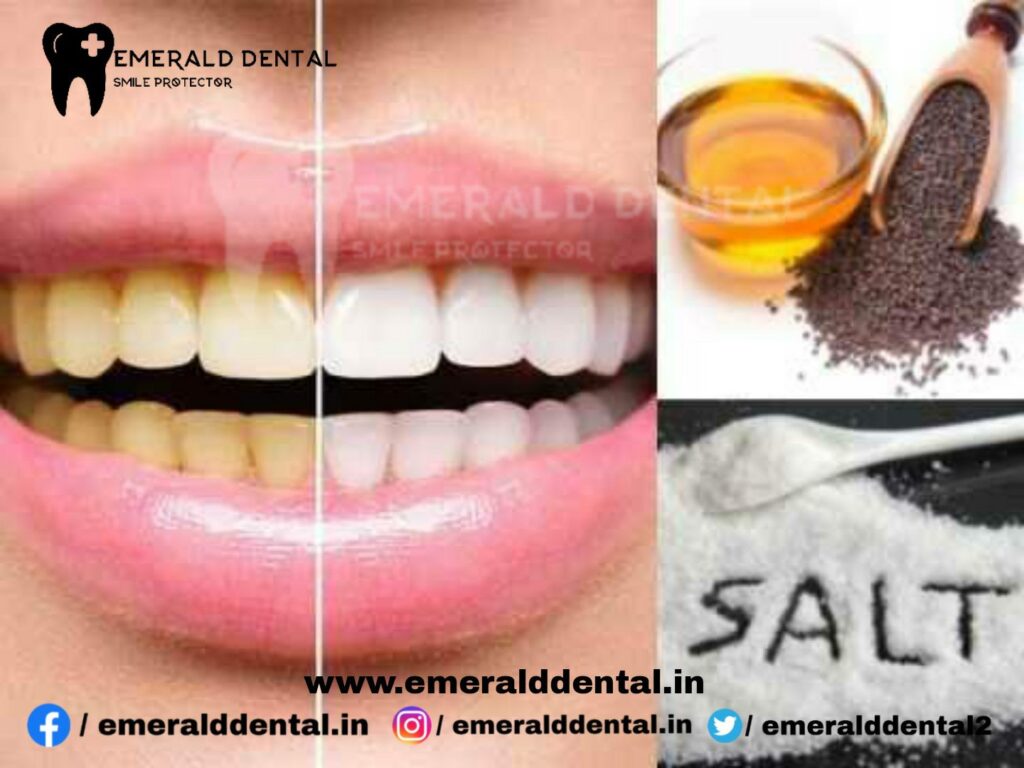The visual layout of the social media ad for Emerald Dental Smile Protector is cleverly organized into two distinct columns for a striking impact. The prominent left column features a side-by-side comparison of a person's smiling mouth. A vertical white line bisects this column, creating a before-and-after effect. On the left side of the line, the teeth appear noticeably yellowed, whereas, on the right side, the same teeth have been transformed to a bright, pristine white, illustrating the results of Emerald Dental's services.

In the top left corner of the ad, the Emerald Dental Smile Protector logo is clearly visible, establishing brand identity. The narrower right column contains two individual images. The top image showcases a natural display of honey with brown seeds and a wooden spoon, possibly hinting at natural ingredients or home remedies. Below it, the black-and-white image artfully displays salt with the word "SALT" spelled out within the granules, adding a unique, eye-catching element.

At the bottom of the ad, viewers can find the website for the dental office along with icons and links for all their social media platforms, making it easy for potential customers to connect and learn more.

Overall, the ad effectively combines vivid visuals and clear, inviting information to attract new clients to Emerald Dental Smile Protector.